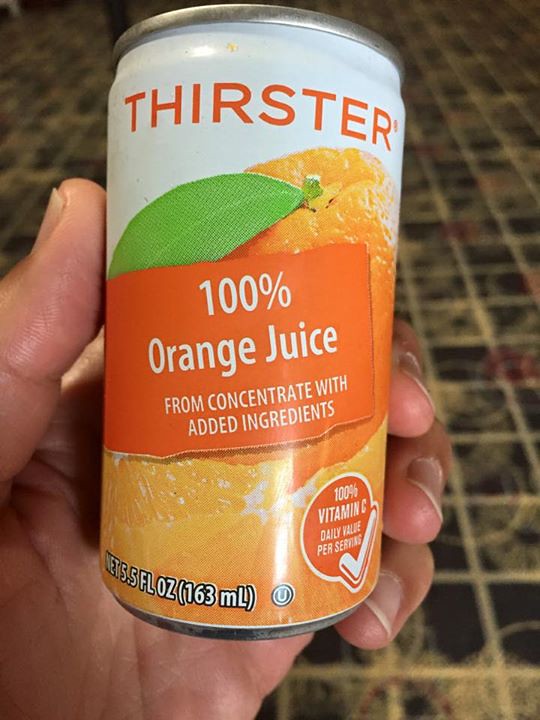This detailed close-up depicts a person's left hand holding a can of Thirster 100% orange juice from concentrate with added ingredients. The can, about the size of a typical soda can, has a net weight of 5.5 fluid ounces (163 milliliters). Its design features a prominent white top with "THIRSTER" in bold orange uppercase letters. Below, there is an image of a whole orange with a green leaf, and a bright orange banner stating "100% orange juice from concentrate with added ingredients." Further down, an image of peeled orange segments is visible. In the right-hand corner, a circle with a white check mark declares "100% vitamin C daily value per serving." Additionally, there's a small circle with a U, indicating certification, likely Kosher. The person's thumb is positioned on the right side of the can, with their fingers wrapping around it, against a backdrop that might include some flooring.